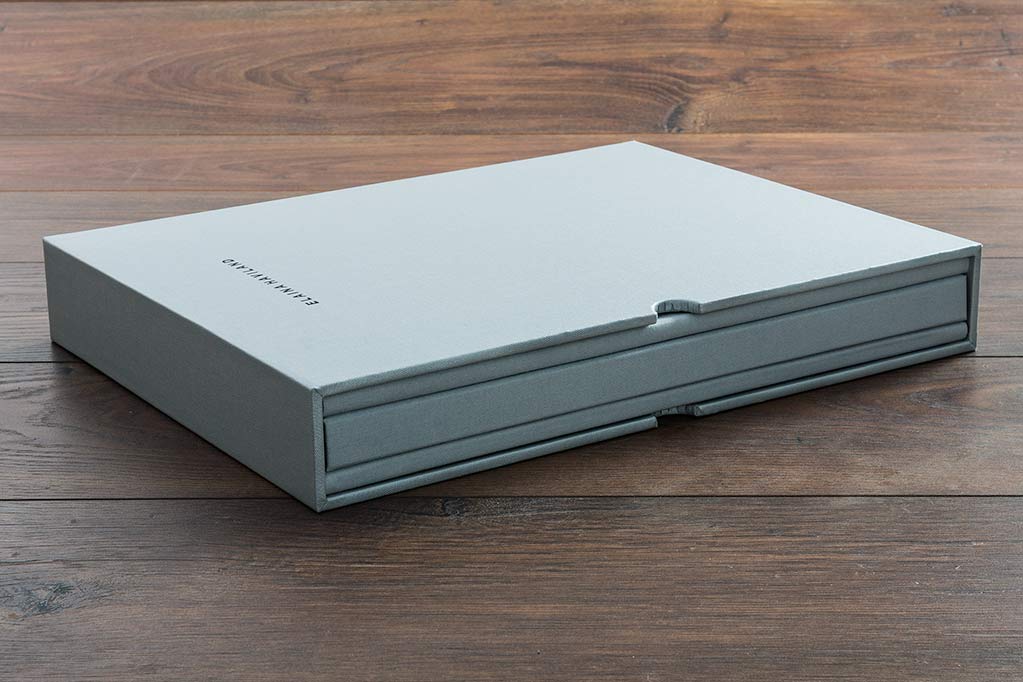This close-up image captures a still life of a light blue or faint gray rectangular sleeve, possibly made of cardboard, resting on a brown, wooden surface that might be a table or a floor. The scene is bright and clear, likely due to natural light. The sleeve houses what appears to be three books of varying thicknesses; a thin book is visible alongside a thicker one and another thin one. On the side of the sleeve, there are small circular cutouts designed for easy removal of the books. The top of the sleeve features black lettering that appears to read "Elena Haviland," although it is oriented in the opposite direction, making it difficult to decipher. The overall image is sharp, with no other objects visible in the frame, focusing solely on the sleek, protective cover and the items within it.